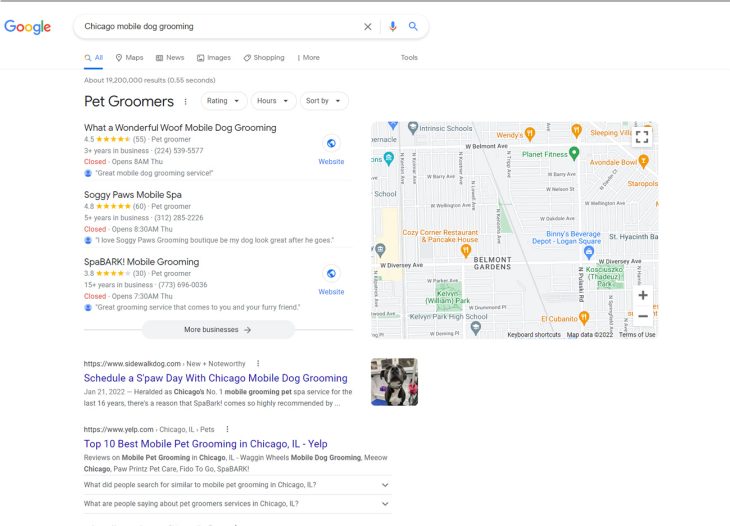The image depicts a Google search results page. In the upper left corner, the Google logo is visible. To the right of the logo is the Google search bar, which contains the query "Chicago mobile dog grooming." Below the search bar, there is a menu bar that includes options such as "All," "Maps," "News," "Images," "Shopping," and "More." The "All" tab is currently highlighted with a horizontal bar beneath it.

The search results are as follows:
1. The top result is "What a Wonderful Wolf Mobile Dog Grooming," which has a rating of 4.5 stars. The listing indicates that the business is currently closed and will open at 8 a.m. on Thursday.
2. The second result is for "Soggy Paws Mobile Spa."
3. The third result is "Spa Bark Mobile Grooming."

To the right of the search results, there is a map highlighting the Belmont Gardens area. The map also shows several pins indicating the locations of other businesses, including restaurants and shopping venues.